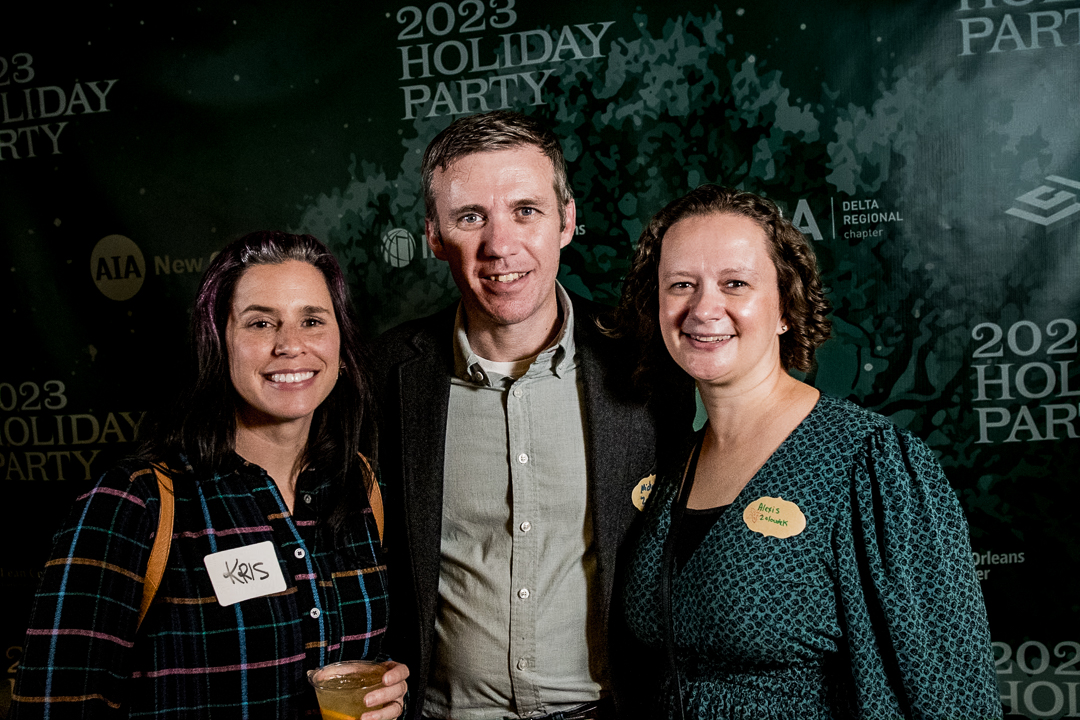The image captures a lively moment from the 2023 holiday party hosted by the AIA Delta Regional Chapter, as indicated by the text on the decorative camouflage-inspired green background. In the center, three individuals are closely grouped, all smiling warmly towards the camera. The woman to the left, identified as Chris by her name tag, has long, dark dyed hair and wears a black button-up shirt with blue, pink, and yellow grid-like stripes. She complements her outfit with brown-strapped backpack and holds a clear glass with ice and a brown liquid. 

Flanking Chris is a man dressed in a dark grey blazer over a green collared button-up shirt, layered with a white t-shirt. He has short hair and exudes a friendly demeanor. 

To the right stands another woman in a long-sleeved green dress with a black undershirt. Her short brown hair frames her face as she looks directly into the camera. Though her name tag is illegible, its distinctive brown sticker with green text adds a subtle detail to her ensemble. The three attendees, amidst this festive backdrop, encapsulate the camaraderie and joy of the event.